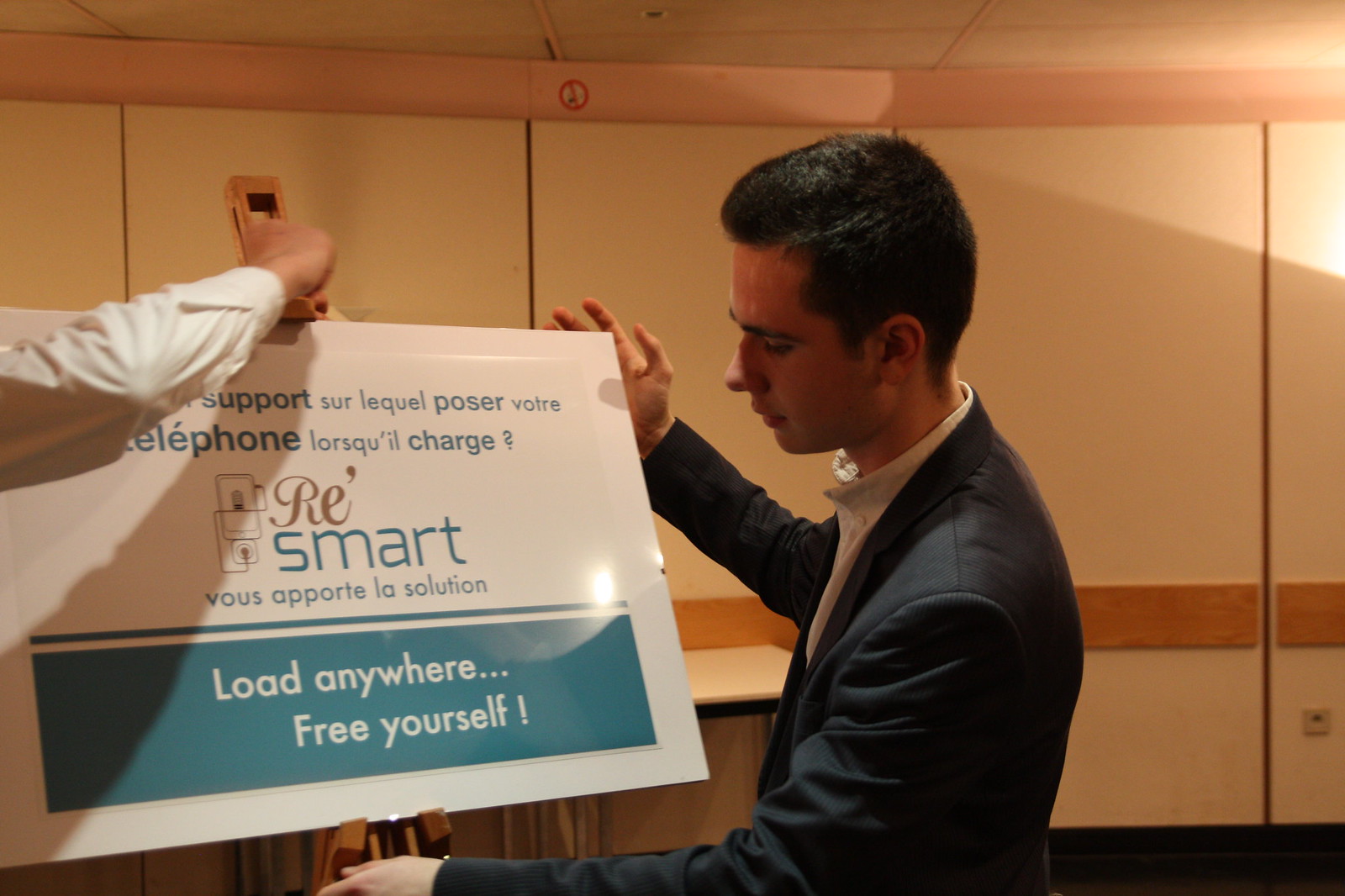The photograph captures a scene at chest level of a man in a black suit and another person, distinguishable only by his white-shirted right arm, working together to position a white sign on a small wooden easel. The sign contains text in blue and light brown, starting with "Support Sir Leequell Poser Votre" and "Telephone Foscui Il Charge," though parts are obscured by the man's arm. Further down in light brown text, it says "RE," followed by "Smart" in blue, and "Vos Apporte La Solution." At the bottom, it states, "Load Anywhere… Free Yourself" in white text. The background features a white wall with a pink border, as well as a "No Smoking" sign visible on the back wall.